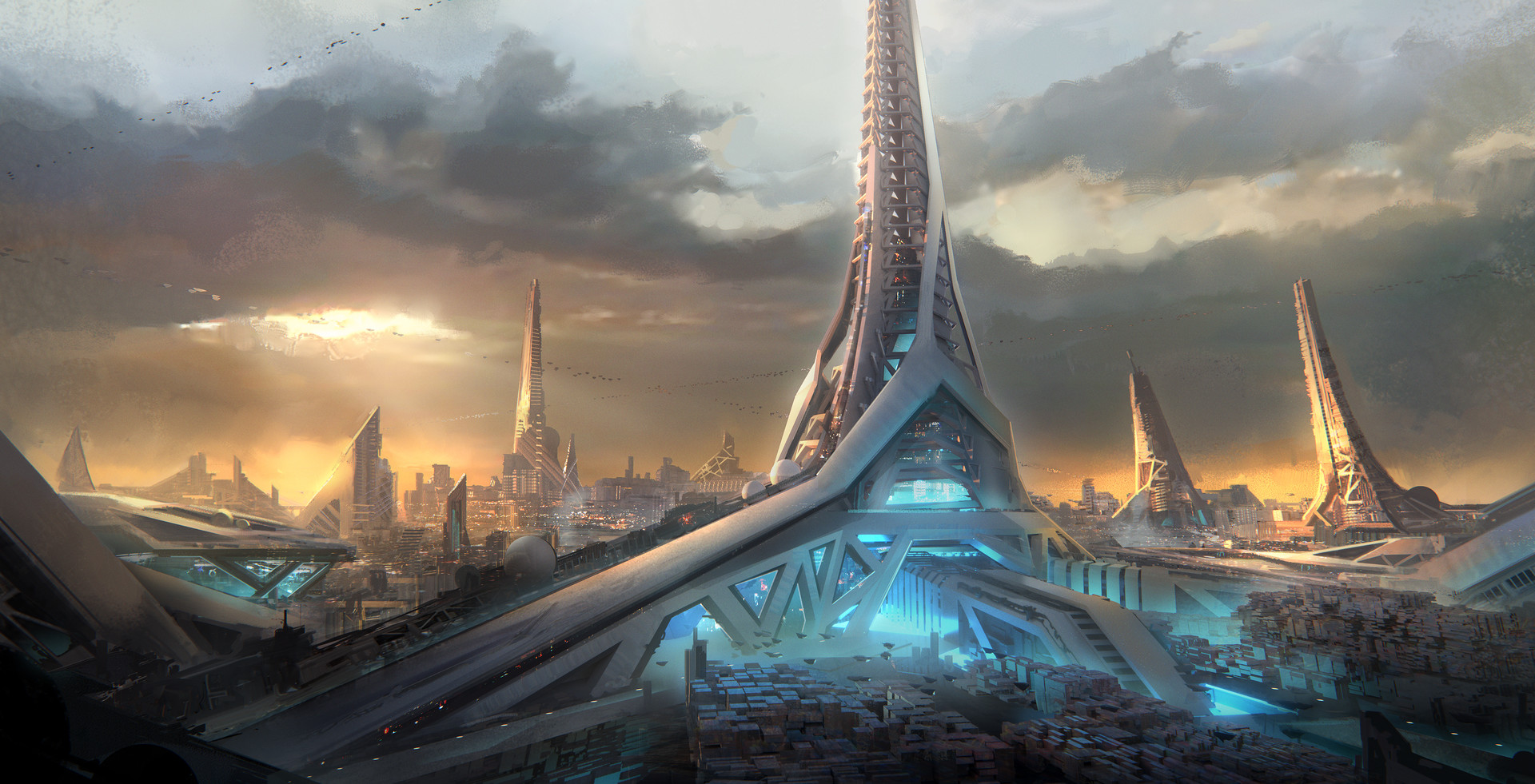The image is a detailed, digitized artwork depicting a futuristic city on a different planet. The central elements are exceedingly tall, spire-like structures and towers that soar vertically into a gray, cloud-filled sky with occasional beams of sunlight piercing through. These immense structures, primarily gray or silver, are adorned with numerous windows and encircled by walkways, suggestive of possible living quarters. At the base of the foremost tower, there is a captivating blue light, casting an ethereal glow in the otherwise stark environment. Surrounding this central tower are piles of boxes and a road leading into it, hinting at bustling activity below the towering spires. In the background, three more grandiose towers loom, alongside smaller buildings and additional towers, contributing to the vast, sprawling metropolis. On the left, low in the image, a spaceship appears to be descending towards the cityscape, adding to the sci-fi ambiance. The sky is predominantly dark gray with scattered black clouds, through which the sun's yellow light occasionally breaks, reflecting off the spires and adding depth to the scene. The artwork skillfully blends digital and watercolor techniques, evoking a sense of futuristic wonder and complexity.